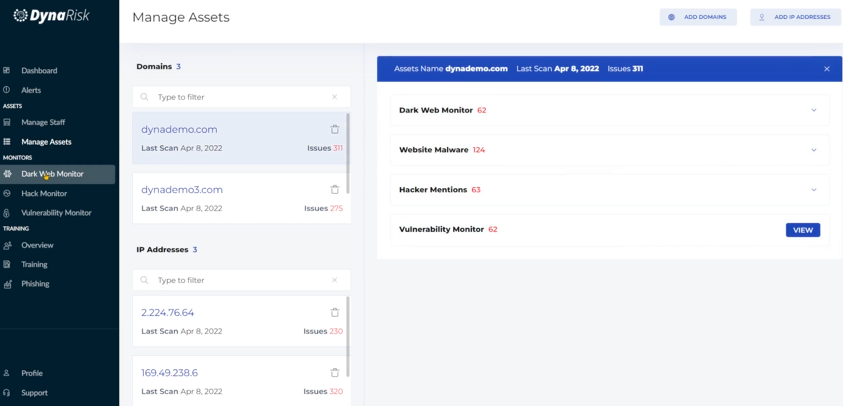The image depicts a detailed interface of a cybersecurity monitoring platform named "DynaRisk." The left-hand side of the interface features a column set against a navy blue background. At the top of the column, "Dyna" is displayed in bright, bold white font, while "RISK" follows in regular white font; both parts of the name incorporate capital letters for 'D' and 'R,' respectively, presenting a unified brand name, "DynaRisk." Adjacent to the name is a small logo.

Beneath the logo are various categorized options indicated by icons. The first section, labeled "Assets," includes "Dashboard," "Alerts," "Manage Stuff," and "Manage Assets." Further down, under the "Monitors" category, are "Dark Web Monitor," "Hack Monitor," and "Vulnerability Monitor." Another category, with an unclear header, lists "Overview," "Training," and what appears to be "Phishing."

To the right of this column, the interface shows the words "Manage Assets" in gray font. At the top-right corner, there are two blue buttons: one reading "Add Domains" and the other possibly reading "Add Addresses."

Returning to the left section of the image, bold black text indicates a section titled "Domains," accompanied by the number three. A search bar labeled "Type to Filter" allows for specific searches. Underneath, the domain "dynadermo.com" is listed twice along with the dates of their scans. Additionally, "IP Addresses" is shown in bold font followed by some specific entries.

In the middle of the interface, a prominent bright blue horizontal rectangular area displays the text "dynadermo.com" in white font, although the font is too small to be entirely legible. Directly below, the text "Dark Web Monitor," "Website Malware," "Hacker Mentions," and "Vulnerability Monitor" appear in bold black font. Each of these options includes a blue "VIEW" button in white, capitalized text to the right.

Overall, the image provides a comprehensive view of the DynaRisk dashboard, highlighting various monitoring and management features available within the platform.